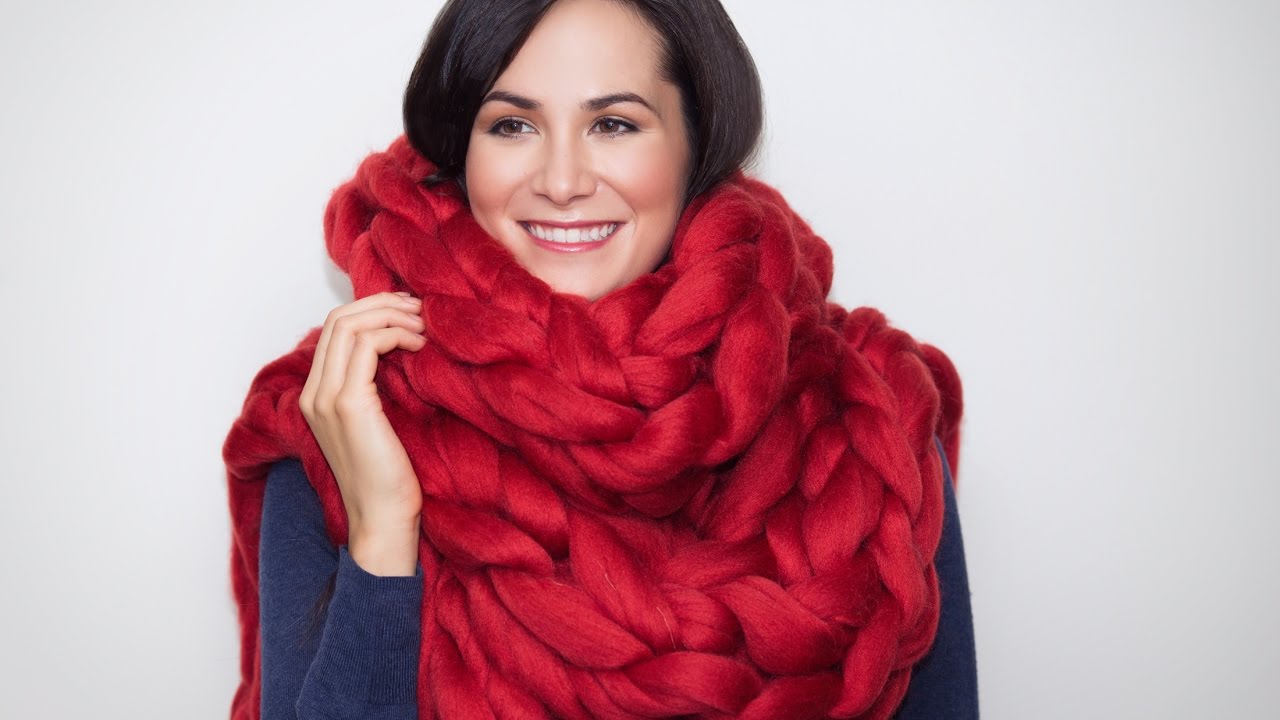In this detailed photograph, a woman with dark brunette hair and dark brown eyes is smiling warmly while looking slightly to her right. She is seen from the chest up, dressed in a long-sleeved navy blue shirt. The standout feature is her large, braided red scarf, which wraps snugly around her neck and drapes elegantly over her shoulders, covering her entire chest and extending down her back. Her right hand is gently holding onto the scarf, while her left arm rests by her side. She has a light tan complexion and is wearing makeup that includes rosy cheeks and a subtle pinkish-red lipstick. The background is a neutral light gray, providing a clean and simple backdrop that emphasizes her cheerful expression and distinctive red scarf. She appears to be in her late 30s to early 40s.